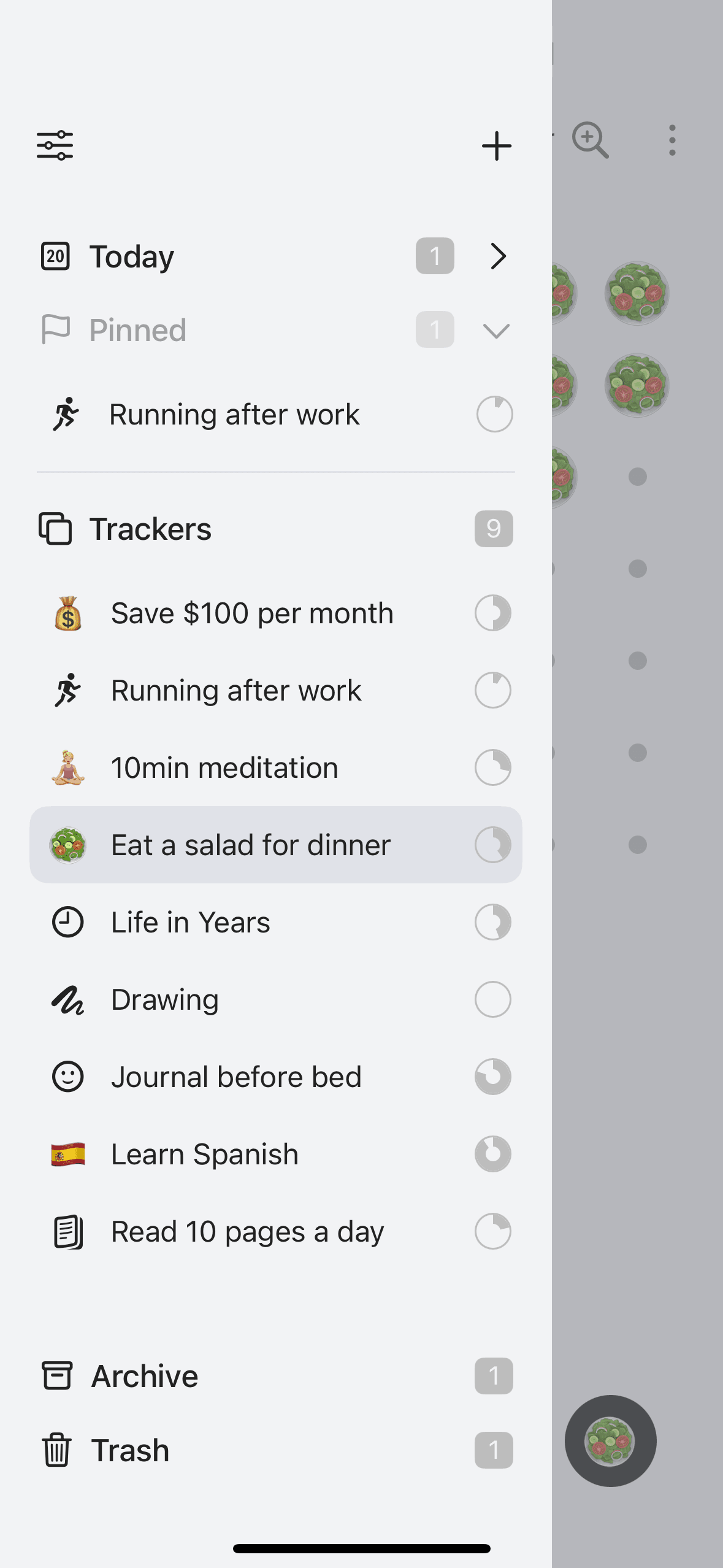A screenshot from a cellphone display showcases a well-organized list of tasks and trackers, each accompanied by unique icons. At the very top, the date is marked with "Today" and beside it is the section "Pinned" with a flag icon denoting pinned tasks. Below these is a heading labeled "Trackers" in faint gray, followed by a list of tasks. 

1. **"Today"**: The number 20 is displayed.
2. **"Pinned"**: A flag icon depicting a pinned item.
3. **"Running after work"**: Represented by a stick figure running icon.

A thin gray line separates these from the main task list:

1. **"Save $100 per month"**: Accompanied by an image of a money bag.
2. **"Running after work"**: Illustrated with a stick figure running.
3. **"10-minute meditation"**: A person sitting cross-legged.
4. **"Eat a salad for dinner"**: A bowl of salad.
5. **"Life in years"**: A clock icon.
6. **"Drawing"**: An abstract scribble.
7. **"Journal before bed"**: A smiling face icon.
8. **"Learn Spanish"**: The Spanish flag with its red, yellow, and red colors.
9. **"Read 10 pages a day"**: An icon of an open book.

At the bottom of the list, separated by some space:

1. **"Archive"**
2. **"Trash"**: Featuring an icon of a trash can.